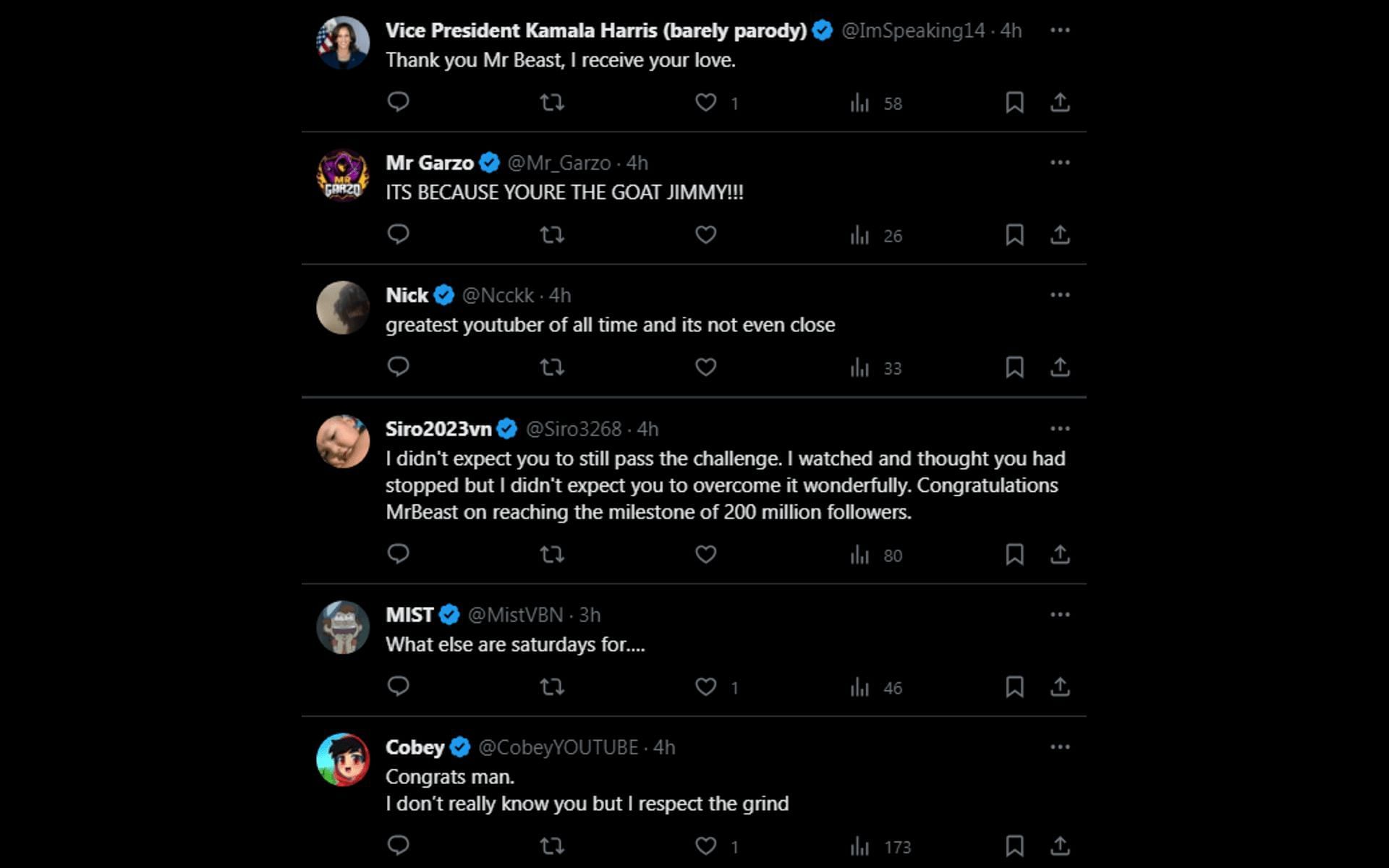The image showcases a series of Twitter posts displayed in dark mode, characterized by a black background and white text, with all accounts marked with blue checkmarks, indicating verified users.

- The first tweet is from a parody account of Vice President Kamala Harris, stating: "Thank you, Mr. Beast. I receive your love."
  
- Below it, a tweet from Mr. Garza enthusiastically reads: "It's because you're a goat, Jimmy!!!"
  
- The next tweet by Nick declares: "Greatest YouTuber of all time, and it's not even close."

- Following that, a user named Zero2023VN reflects on Mr. Beast's perseverance: "I didn't expect you to still pass the challenge I watched and thought you had stopped, but I didn't expect you to overcome it wonderfully. Congratulations, Mr. Beast, on reaching the milestone of 20 million followers."

- The succeeding tweet from Missed enigmatically states: "What else are Saturdays for..."

- Lastly, Kobe, a user unfamiliar with Mr. Beast, offers respect: "Congrats, man. I don't really know you, but I respect the grind."

This collection of tweets celebrates Mr. Beast's achievement of reaching 20 million followers, with various users, both sincere and parody, expressing their admiration and congratulations.